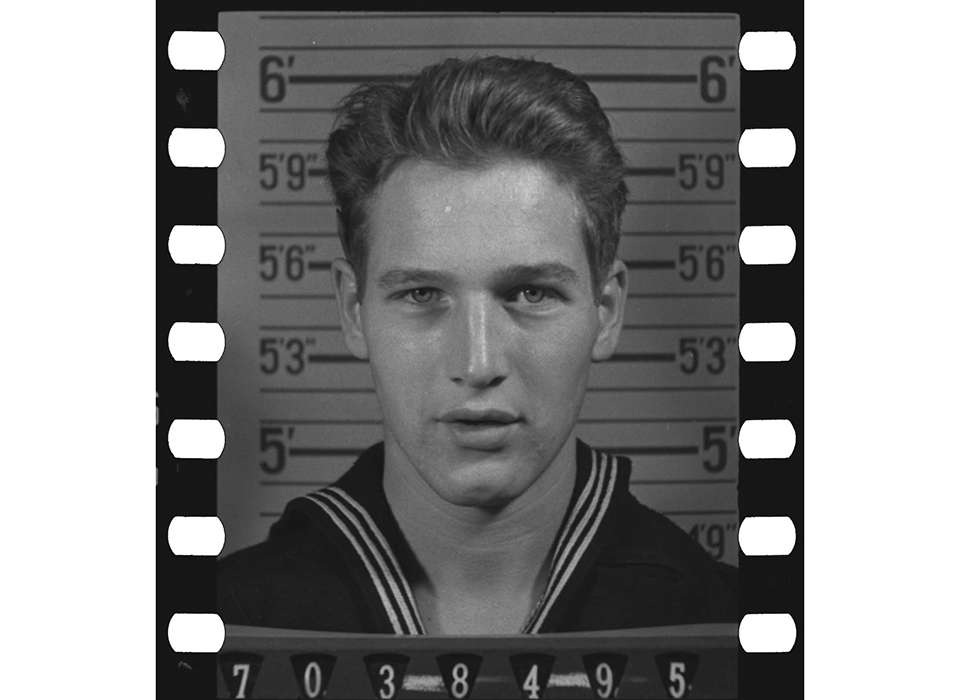This black-and-white photograph appears to be a scanned 35mm film negative. It captures a man in what looks like an old-style navy uniform, possibly indicating he was set to join the navy. His hair is slicked back, and he stands against a wall marked with height indicators, showing measurements from 4'9" to 6'. His hair reaches slightly above the 6' mark. The backdrop and his head and shoulders framing resemble a classic mug shot style. The image includes visible imperfections typical of film, such as dust and scratches. There are vertical rows of white, capsule-shaped dots on the left and right sides, which are the film's sprocket holes. At the bottom of the photo, the numbers "7038495" are printed, potentially an identification number. The man is looking directly at the camera with a slight smile on his face.